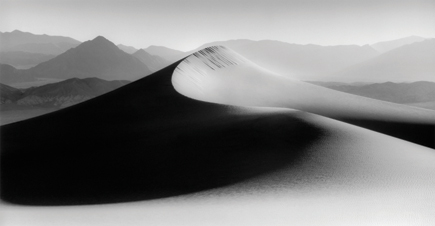This black-and-white photograph captures a dramatic desert landscape, masterfully showcasing the play of light and shadow, or chiaroscuro, across expansive sand dunes. Dominating the foreground is a massive wavy sand dune, its pronounced peak creating a swirling effect that curves gracefully to the lower right corner. The dune's left side is steeped in deep shadow, contrasting starkly with the bright, illuminated sections, creating an almost yin-yang effect. Further back, the dunes become smaller and blurrier, extending towards a hazy horizon where they meet a featureless, grayish-white sky. Jagged, rocky mountains, reminiscent of those found in deserts such as the Sahara, Gobi, or Death Valley, are stacked in the background, adding to the image's atmospheric depth. The overall effect is a stunning artistic composition, emphasizing the raw, rugged beauty of the desert terrain.